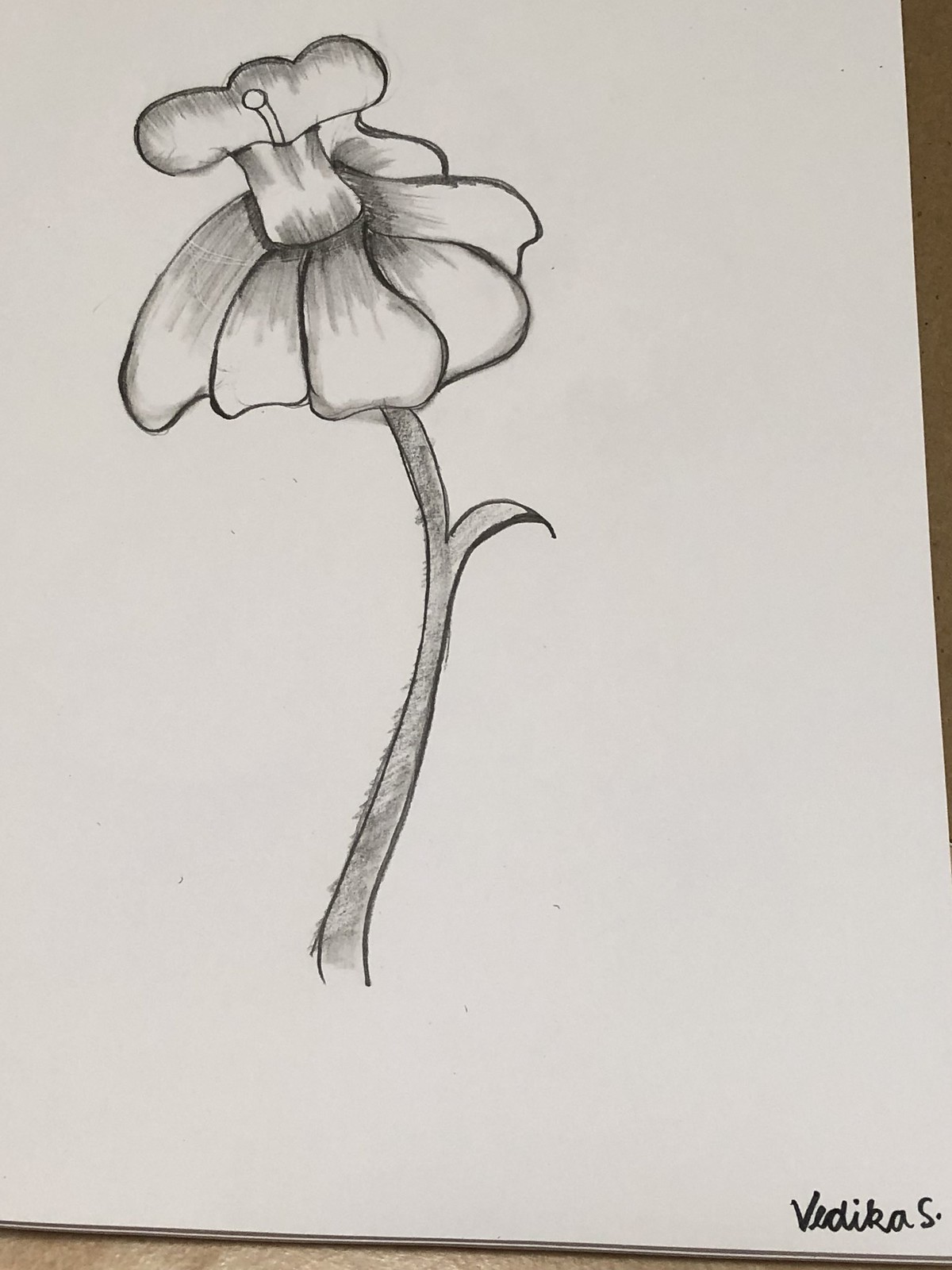A detailed, cleaned-up version of the caption could be:

"Captured from a top-down perspective, this image showcases a beautifully detailed pencil drawing of a flower on a white sheet of paper, which appears to be part of a notepad resting on a wooden surface. The drawing features a delicate stem with a small, shaded leaf branching off. The flower is composed of several petals, which gracefully droop downward and towards the bottom of the image. Notably, the upper sections of these petals are shaded, whereas the lower parts remain unshaded, creating a dynamic contrast. At the top of the flower, an intricate structure unfolds, reminiscent of the iconic shape of an atomic bomb explosion. Surrounding this central feature are additional petals, while a prominent, completely white stamen or stem extends from its center, adding a striking focal point to the drawing."